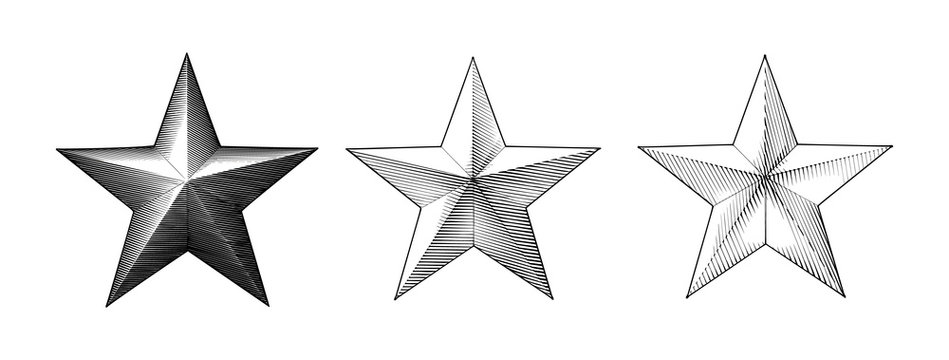This is a detailed black-and-white illustration set against a plain white background featuring three five-pointed stars aligned horizontally. Each star resembles a person with arms spread out, legs beneath them, and a point representing the head on top. The stars appear to be sketched with a pencil, characterized by fine lines and varying degrees of shading. The star on the left is the darkest, heavily shaded with visible pencil strokes suggesting light shining from the top left. The middle star is lighter, with more visible lines and less shading compared to the first. The star on the right is the lightest of the trio, with minimal shading but still displaying some black lines. Each star appears to be in relief, giving a subtle three-dimensional effect reflecting directional lighting.